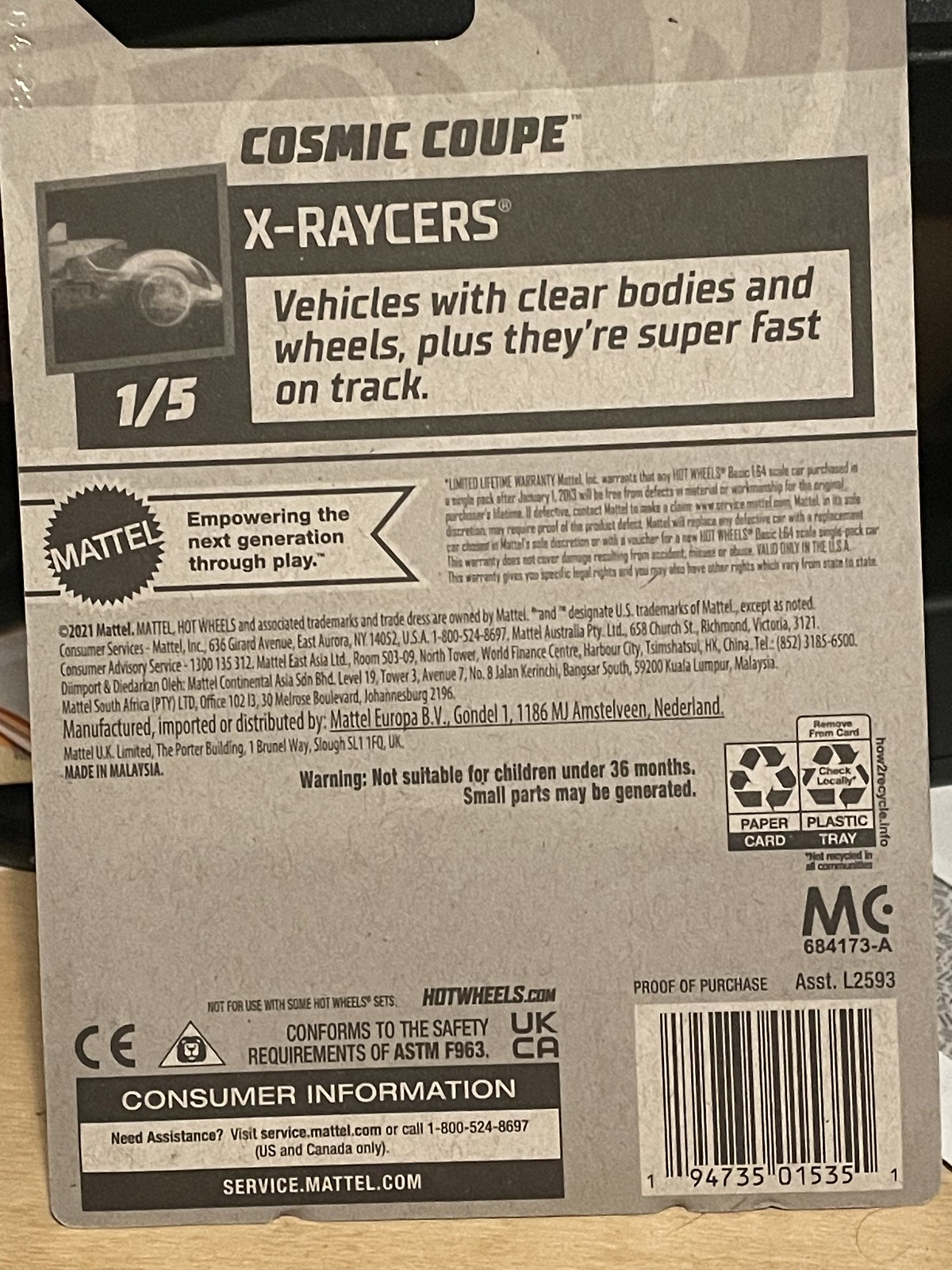The image captures the back of a toy vehicle package, most likely a matchbox car, made from cardboard. The back is entirely in black and white and features a cutout at the top left for retail display hanging. The color scheme transitions from light gray to very dark gray, almost black. At the top, bold text announces "Cosmic Coop X-Racers" (spelled X-R-A-Y-C-E-R-S), with a subheading that reads "Vehicles with clear bodies and wheels, plus they're super fast on track." Adjacent to this text, there’s a black and white image of the X-Racer labeled "1/5," indicating it is the first in a series of five. Below this image is the distinctive circular Mattel logo, described as a sun with jagged edges. Accompanied by the slogan "Empowering the next generation through play," fine print legal information, addresses, limited warranty, and safety warnings like "Not suitable for children under 36 months, small parts may be generated" can be seen. Additionally, recycling logos for paper, card, and plastic tray, as well as a UPC barcode, are present, along with a mention of the website hotwheels.com. The bottom left section contains consumer information directing users to service.mattel.com for further support.